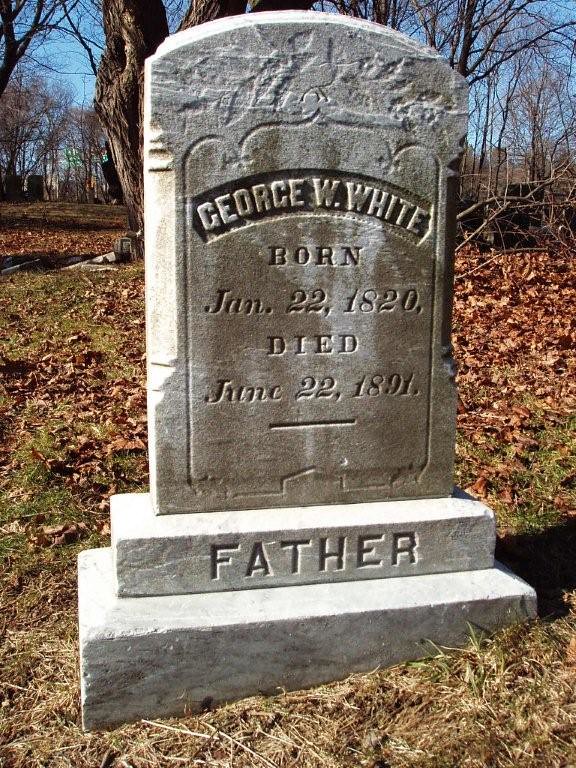The image captures a solitary gray cement tombstone, prominently inscribed with the name "George W. White," who was born on January 22, 1820, and died on June 22, 1891. The word "Father" is engraved at the bottom of the headstone. The name "George W. White" is highlighted against a black background, making it stand out. The tombstone is set against a backdrop of an autumnal scene, with the ground covered in dead leaves and patches of grass. Brown and gray trees, bare of foliage, dominate the background, and the sky is clear. The sunlight streaming from the left casts a shadow to the right of the tombstone. There are no other visible headstones in the shot, giving the image a sense of solitary reverence.